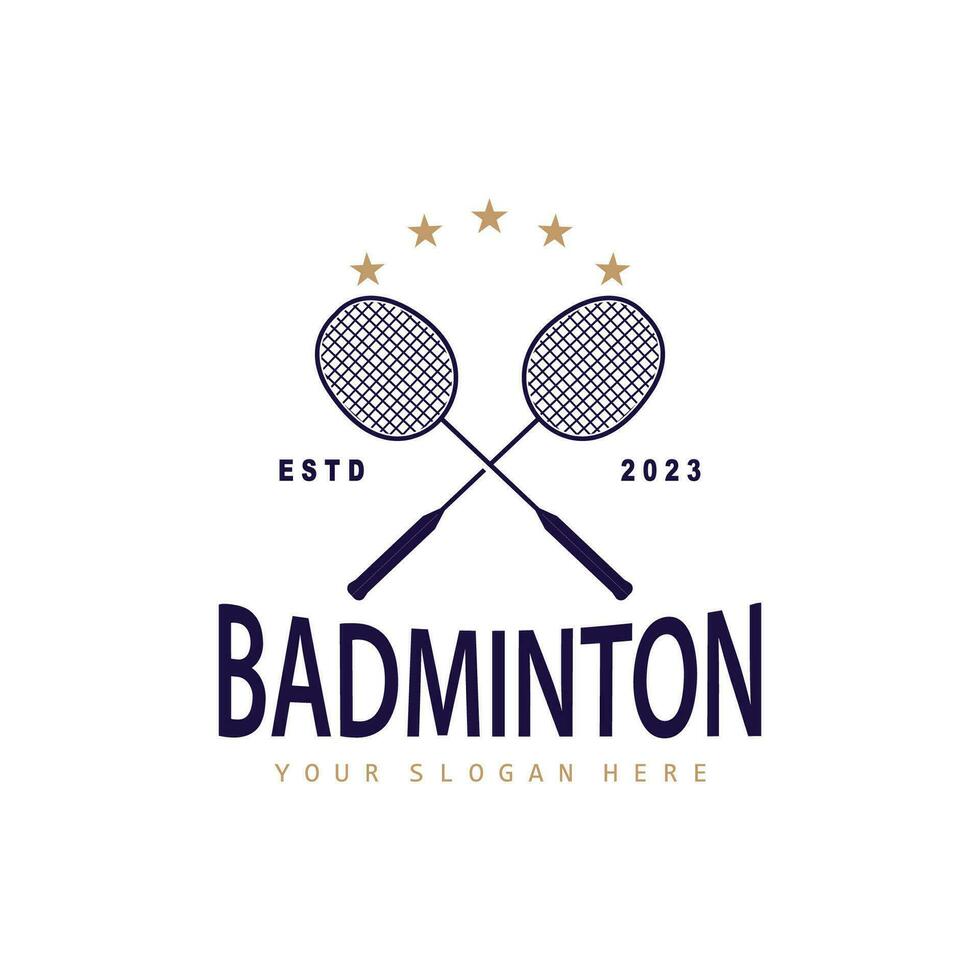This color illustration features a detailed design template with a white background, showcasing a prominent logo centered around the sport of badminton. Central to the design, two blue badminton rackets cross to form an X shape, with clearly defined racket heads and handles. Between the crossed rackets, five gold stars arch gracefully from one racket to the other, forming a symmetrical pattern with one star at the apex and two descending stars on either side. Flanking the rackets, the blue text "ESTD" appears on the left, while "2023" sits on the right, indicating the establishment year. Directly below the rackets, the word "badminton" is written in a bold, stylized blue font. Beneath this, in a simple gray standard font, is placeholder text reading "your slogan here." The color palette primarily includes white, blue, and gold, with the gold stars and the gray slogan text providing complementary accents to the predominantly blue design elements.